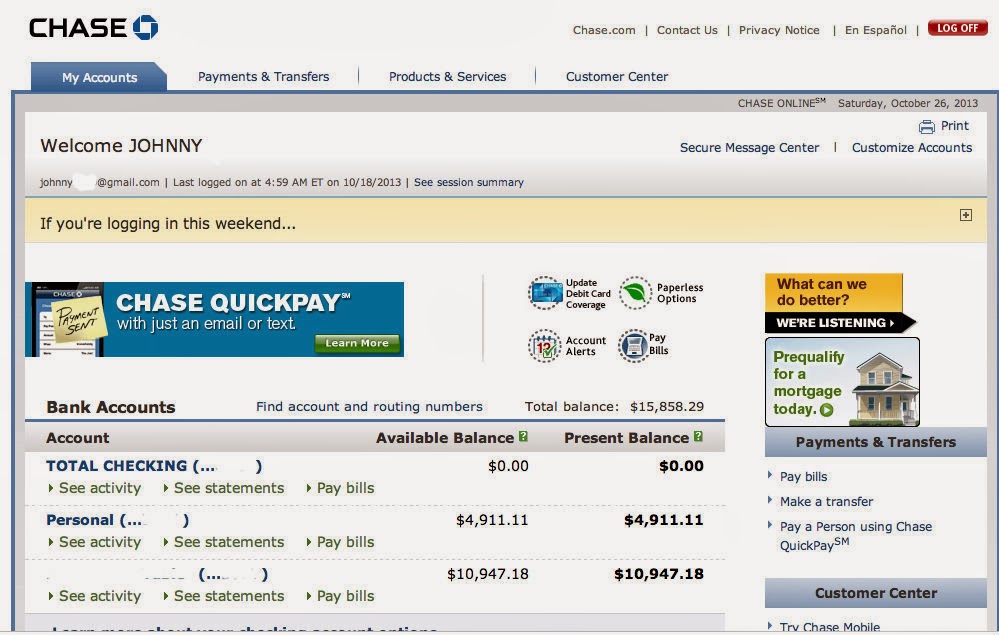A detailed desktop or mobile screen capture of a secure banking interface from Chase is shown. The background of the interface is gray. In the upper left corner, the Chase logo appears in black next to a blue icon. Opposite, in the top right corner, are options labeled "chase.com," "Contact Us," "Privacy Notice," and "En Español," along with a red "Log Off" button. Below the Chase logo, a navigation bar includes "My Accounts," "Payments and Transfers," "Products and Services," and "Customer Center," arranged from left to right with "My Accounts" highlighted. 

An upper border, darker gray in color, holds the text "Chase Online Saturday, October 26, 2013," in the upper right. Returning to a lighter shade, the screen greets the user with "Welcome Johnny," alongside a partially obscured email address ending in gmail.com. The statement "Last logged on at 4:59 A.M. Eastern on October 18, 2013" follows, with a link to a session summary. 

A secure message center and customization options are visible, along with a "Print" button. An advertisement for Chase QuickPay appears with various circular icons detailing its features. Below, Johnny's bank account information displays a total balance of $15,858.29. Detailed sections include options for viewing account activity, downloading statements, and paying bills. A "Payments and Transfer" bar is positioned at the right edge of the screen.